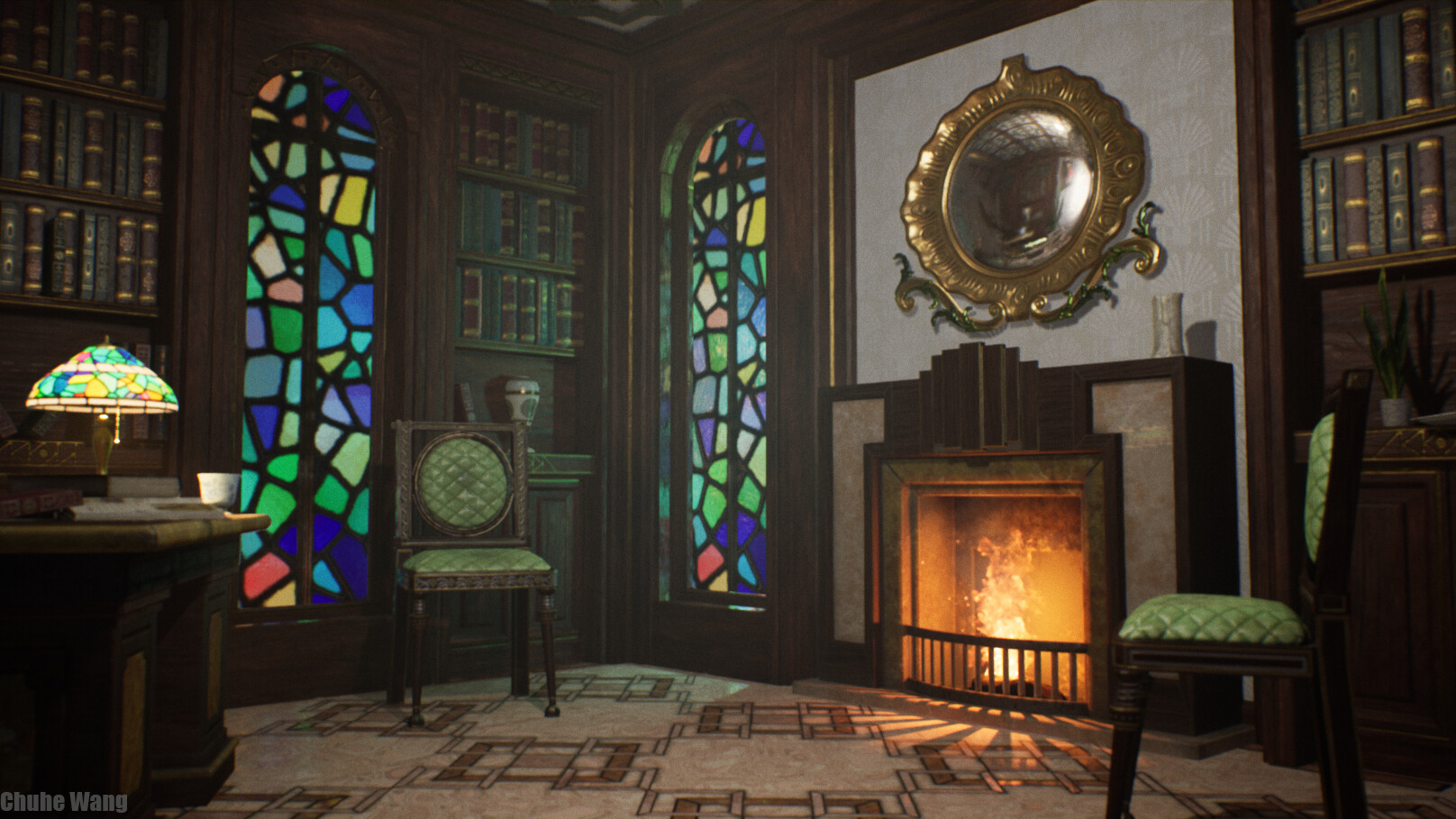The 3D-rendered image depicts an elegant, old-school study room characterized by its rectangular shape. The room's corner features a prominent arched window made of stained glass. Adjacent to this window, on the right side, stands a built-in brown wood shelf filled with an assortment of red, gold, and blue tomes. The bottom shelf of this section showcases a white vase with gold trim. Parallel to this, on the left wall, is another identical stained glass window next to an identical bookshelf. In the bottom left corner of the image is a round wooden desk adorned with a stained-glass style table lamp, which is currently lit, and a white styrofoam cup. On the right side of the room, there is a lit fireplace with a golden mirror above it, flanked on either side by wooden chairs with green cushions. The entire scene is elegantly set on a marble floor with intricate rectangular textures. The study room is a harmonious blend of rich, warm wood, colorful stained glass, and luxurious decorative elements.